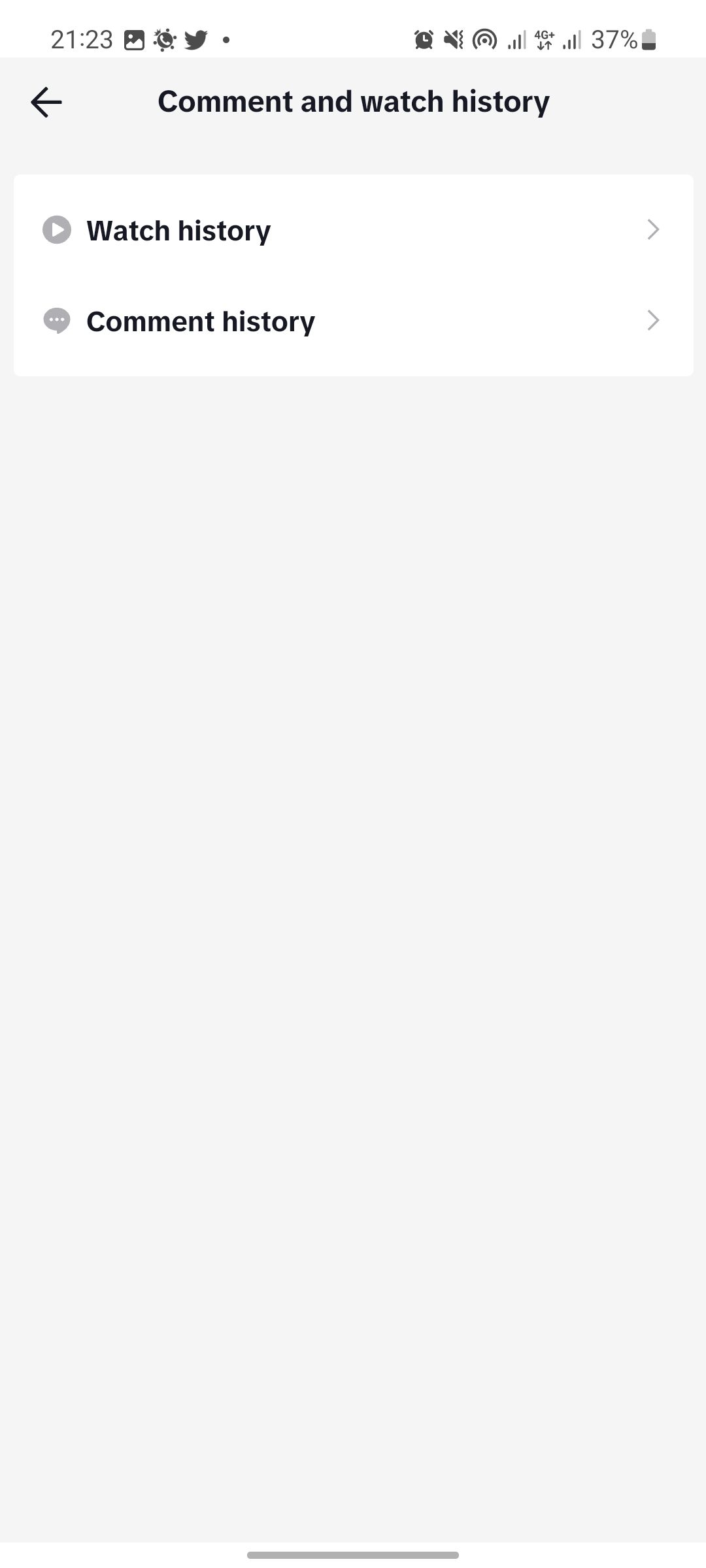The image is a screenshot from a smartphone, exhibiting detailed UI elements. At the top, there's a border approximately one inch high with a gradient of white to gray. Below this, a two-inch white section spans the width of the screen. On the left side of this area, a gray circle encloses a white triangle pointing right, accompanied by the text "Watch history" in black. To its right is a greater-than sign (>).

Underneath, a small comment icon sits next to the text "Comic history" in black, also flanked by a greater-than sign (>) on the far right. From this section extending to the bottom of the screen, the background color shifts to light gray.

Positioned at the bottom center, a dark gray line spans about an inch to the left and right of the midpoint, providing a visual anchor. 

In the top left corner, the time is displayed in military format as "21:23." Adjacent icons include a photo icon, vibrate icon, Twitter icon, alarm clock icon, silence icon, Wi-Fi icon, Internet signal indicator, a "4G" label, and a battery icon indicating 37% charge. The battery icon is partially filled with dark gray (about one-third) while the top portion remains white, outlined by a gray border.